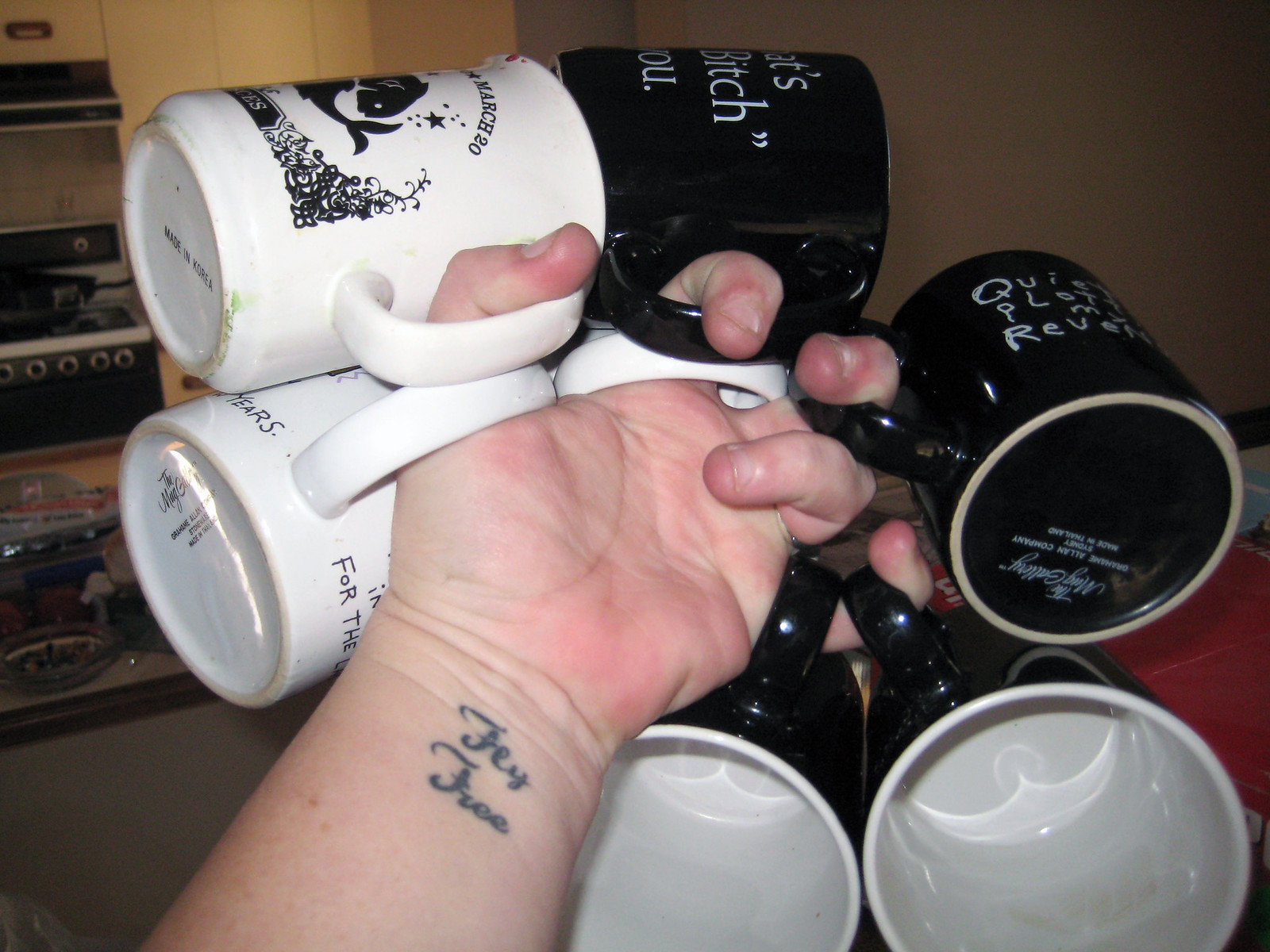In this photograph, a Caucasian man's left hand is precariously grasping six coffee mugs, contorted in a remarkable way to fit them all. Among the mugs, two are white and four are black, each adorned with various logos and text, though the phrases are difficult to decipher due to the arrangement. The mugs are hooked onto his thumb, index finger, middle finger, and pinky, with his fingers curled oddly to maintain the grip. Notably, the man has a tattoo on the inside of his wrist that reads "Fly Free" in stylized script. In the background, the setting appears to be a kitchen, with visible elements such as a stove with a pot on it, a countertop, beige walls, and an ashtray with cigarette butts.